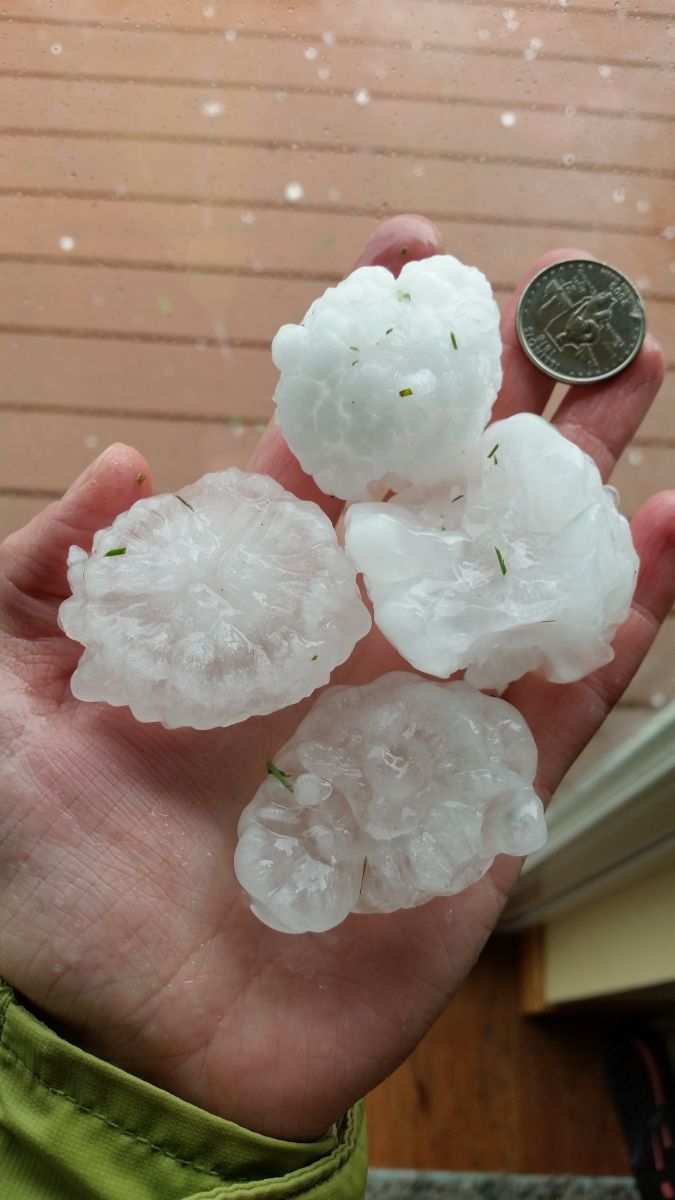In the image, a Caucasian man stands in a doorway with an emphasis on his left hand, which is held palm-up and open. He is wearing a long-sleeved jacket, olive green in color, which covers his wrist. The background reveals a brown wooden floor, the trim of a door, and hints of a brown wooden deck with what appears to be hail scattered across it, suggesting that it might have recently hailed. Inside the house, there's a glimpse of carpet.

The focal point of the photo is the man's hand, which contains five distinct objects: four pieces of large hail and a silver coin, likely used for scale. The hail pieces are white and uniquely shaped, with some appearing translucent and others more solid in color. They also seem to have specks of grass embedded within them. The coin, though not easily identifiable in terms of its exact currency, provides a sense of perspective, indicating the considerable size of the hailstones, as they are larger than the coin itself. The lighting suggests that the photo was taken during the daytime.